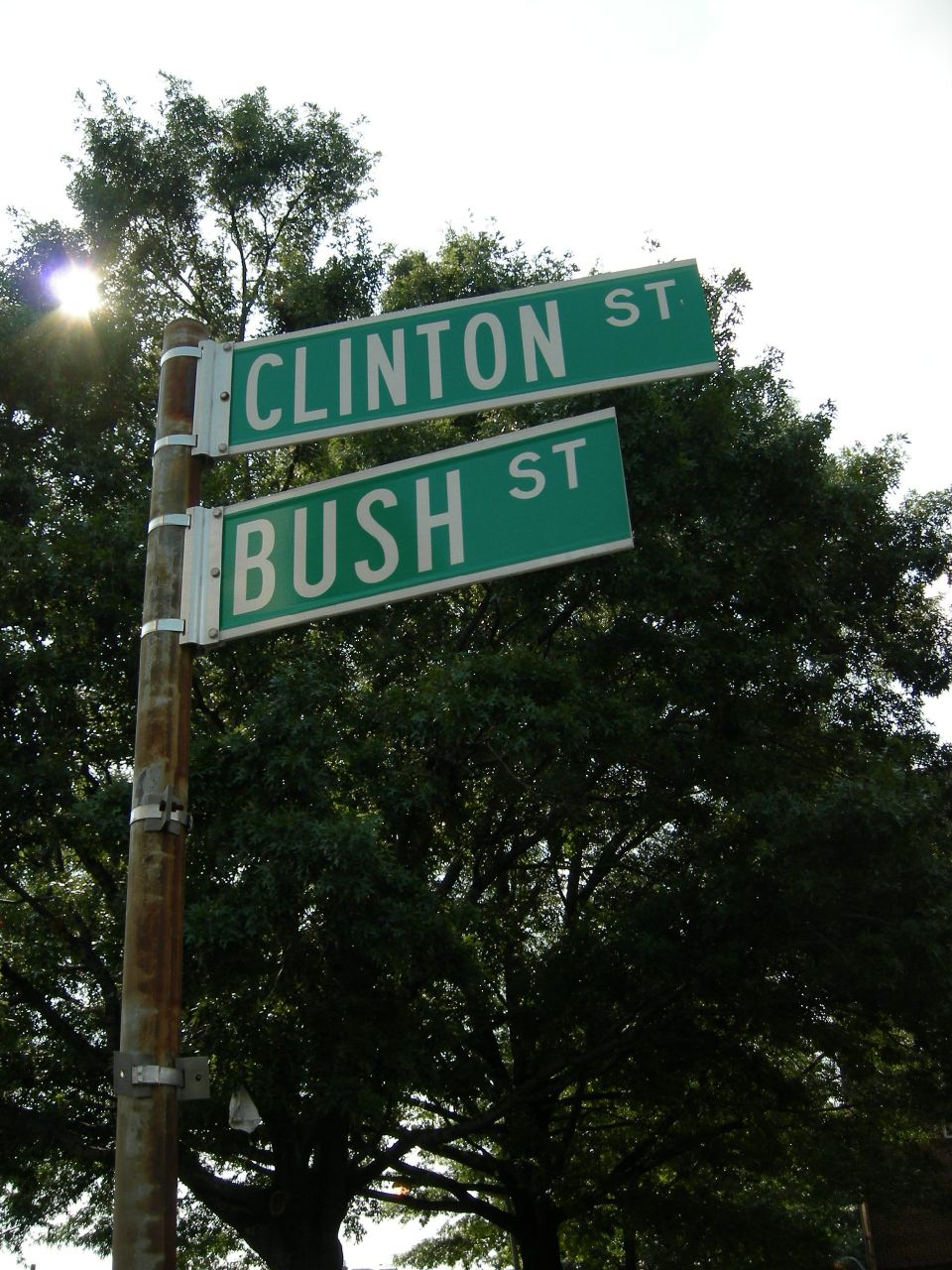In this detailed image, we see two green rectangular street signs for Clinton Street and Bush Street, presumably named after former U.S. presidents, mounted on a grayish-brown pole that appears rusty in places. Both signs, featuring white edges and white lettering, are affixed with silver metal straps and point to the right. Behind these signs stands a cluster of tall trees with dense, dark green leaves, partially blocking the white sky. However, a small gap in the foliage on the top left allows sunlight to peek through, creating a glowing spot. In the distant background, there are hints of a red or dark brown brick building partially obscured by the trees. The perspective of the image suggests it was taken from a low angle, looking upward at the street signs amidst the natural and urban elements.